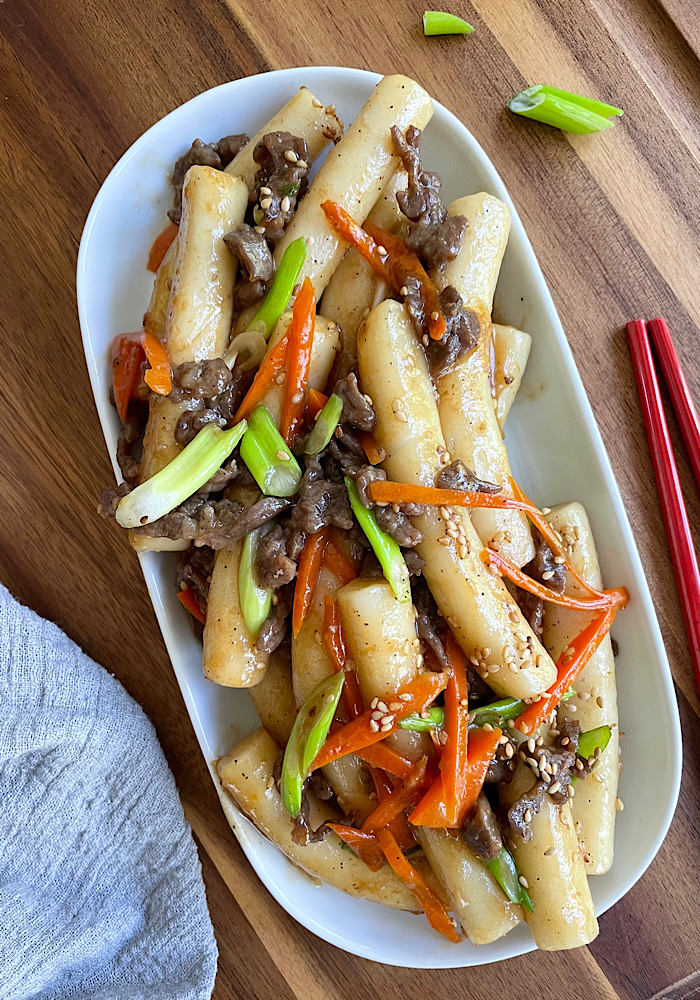This detailed image features an up-close aerial view of a meticulously arranged Asian-style dish, displayed in an oblong, rectangular-shaped white china bowl. The bowl is positioned on a brown wooden tabletop. The dish primarily consists of rigatoni noodles, adorned with vibrant julienned vegetables such as red pepper, carrots, and green onions, as well as sliced mushrooms. A rich, glossy sauce or glaze coats the ingredients, giving them a shiny appearance and implying a flavorful, perhaps slightly sugary, composition. Scattered across the dish are sesame seeds and some pieces of brown shredded meat, reminiscent of the style used in a Philly cheesesteak.

To the right of the bowl, two red wooden chopsticks are visible, partially extending out of the frame, suggesting they may be used to enjoy the meal. Additionally, a small piece of cut green onion is noted on the wooden tabletop, having fallen out of the bowl, adding a casual touch to the presentation. On the bottom left side of the image, a white linen cloth is placed, possibly a napkin or dishcloth, contributing to the overall aesthetic. The carefully arranged vegetables and the clean, deliberate composition suggest that this image could be an advertisement for a restaurant or a high-quality, home-cooked meal meant to showcase culinary skill and presentation.